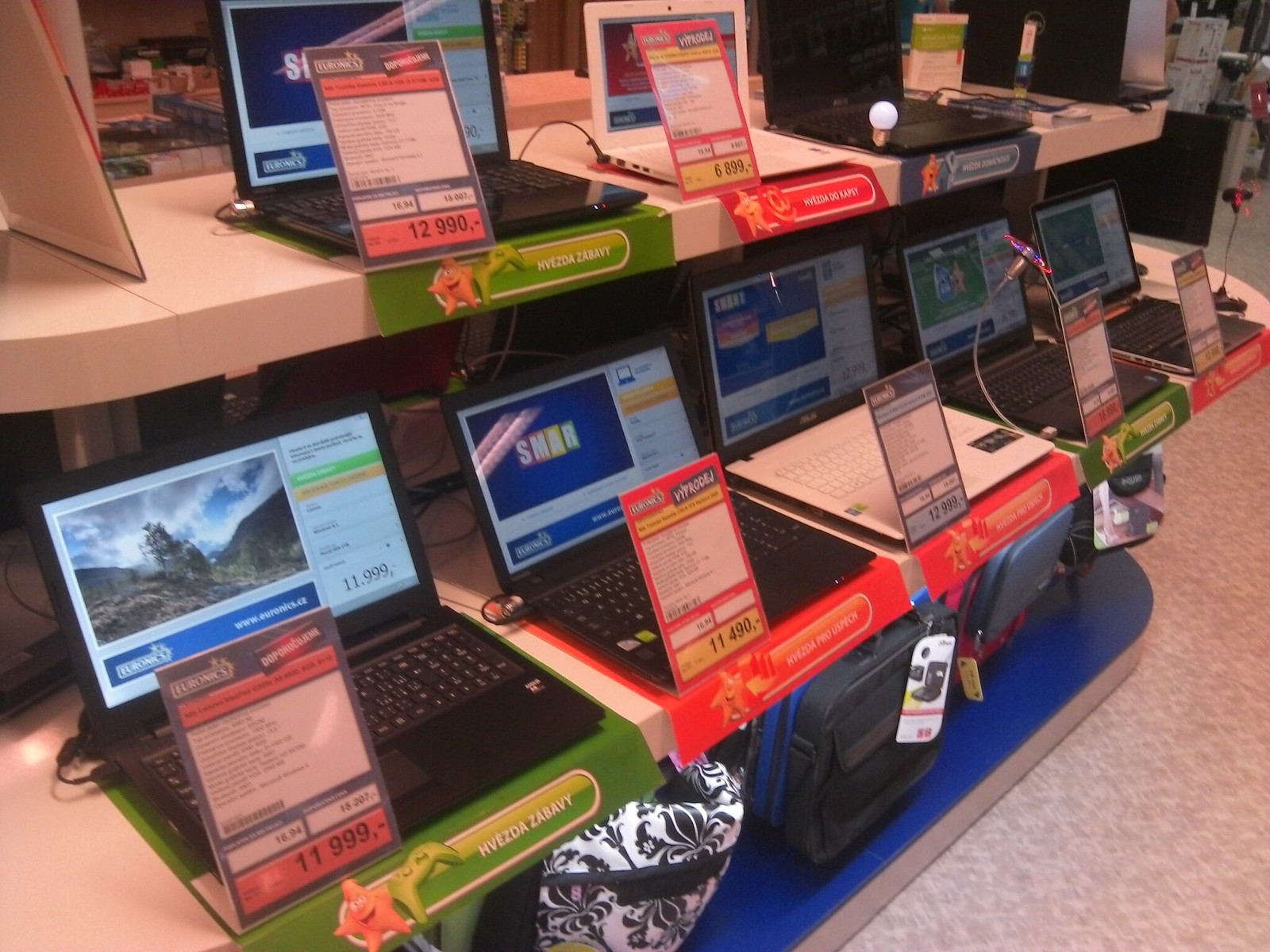The photograph captures a scene inside an electronics store featuring a tiered oval display table with a blue base, showcasing a variety of laptops. The store's floor is white marbled with shades of gray interwoven throughout. The table has three tiers: 

1. **Bottom Tier**: Positioned almost at ground level, this blue-based tier hosts several laptop carrying cases in various designs and colors, including black and white.
2. **Middle Tier**: About waist-high, this tier displays five laptops in different colors (primarily black and silver). The laptops are open and powered on, each accompanied by a brochure-style price tag, indicating prices in a foreign currency.
3. **Top Tier**: Similar in design to the middle tier, this shelf features three laptops, also in a mix of black and white. Each laptop is open with its screen active, and like the middle level, each has a price and information plaque displayed in front.

The image emphasizes the organized layout and the variety of electronics and accessories available for sale, suggesting a modern yet somewhat old-school aesthetic in the laptop designs. All devices are set up to showcase their screens and key features to potential customers, reflecting the meticulous display standards of the store.